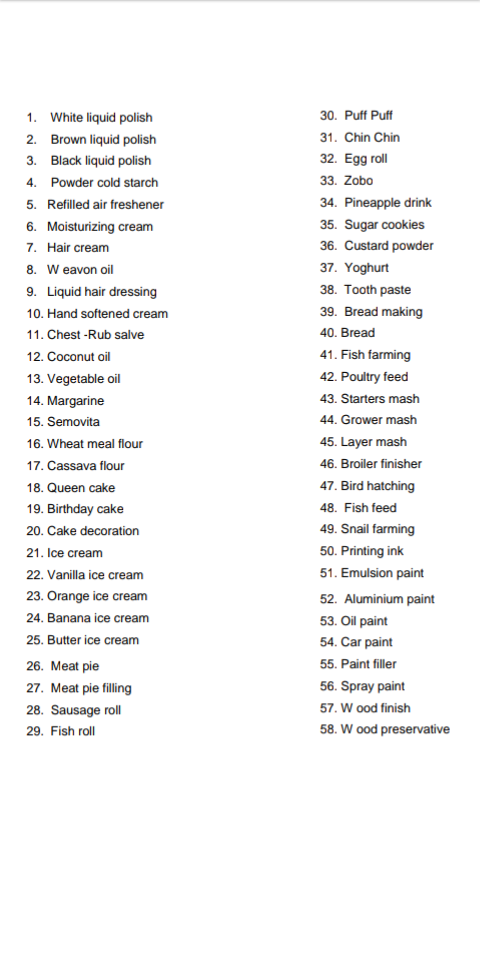This image is a cropped screenshot of a text-based list, displayed in two numbered columns against a white background. The left column includes numbers 1 through 29, while the right column lists numbers 30 through 58. The text is rendered in a small black font. At the top, a thin gray horizontal line spans the width of the image, and just beneath it lies a white blank space before the list begins.

Here is the detailed list from the left column:
1. White liquid polish
2. Brown liquid polish
3. Black liquid polish
4. Powder cold starch
5. Refilled air freshener
6. Moisturizing cream
7. Hair cream
8. W even oil
9. Liquid hair dressing
10. Softened cream
11. Chest rub salve
12. Coconut oil
13. Vegetable oil
14. Margarine
15. Semovita
16. Wheat meal flour
17. Cassava flour
18. Queen cake
19. Birthday cake
20. Cake decoration
21. Ice cream
22. Vanilla ice cream
23. Orange ice cream
24. Banana ice cream
25. Butter ice cream
26. Meat pie
27. Meat pie filling
28. Sausage roll
29. Fish roll

The remainder of the list, numbered 30 through 58, is included in the right column, which has been cropped out in this screenshot. The simplistic and utilitarian design focuses attention on the clearly itemized entries.